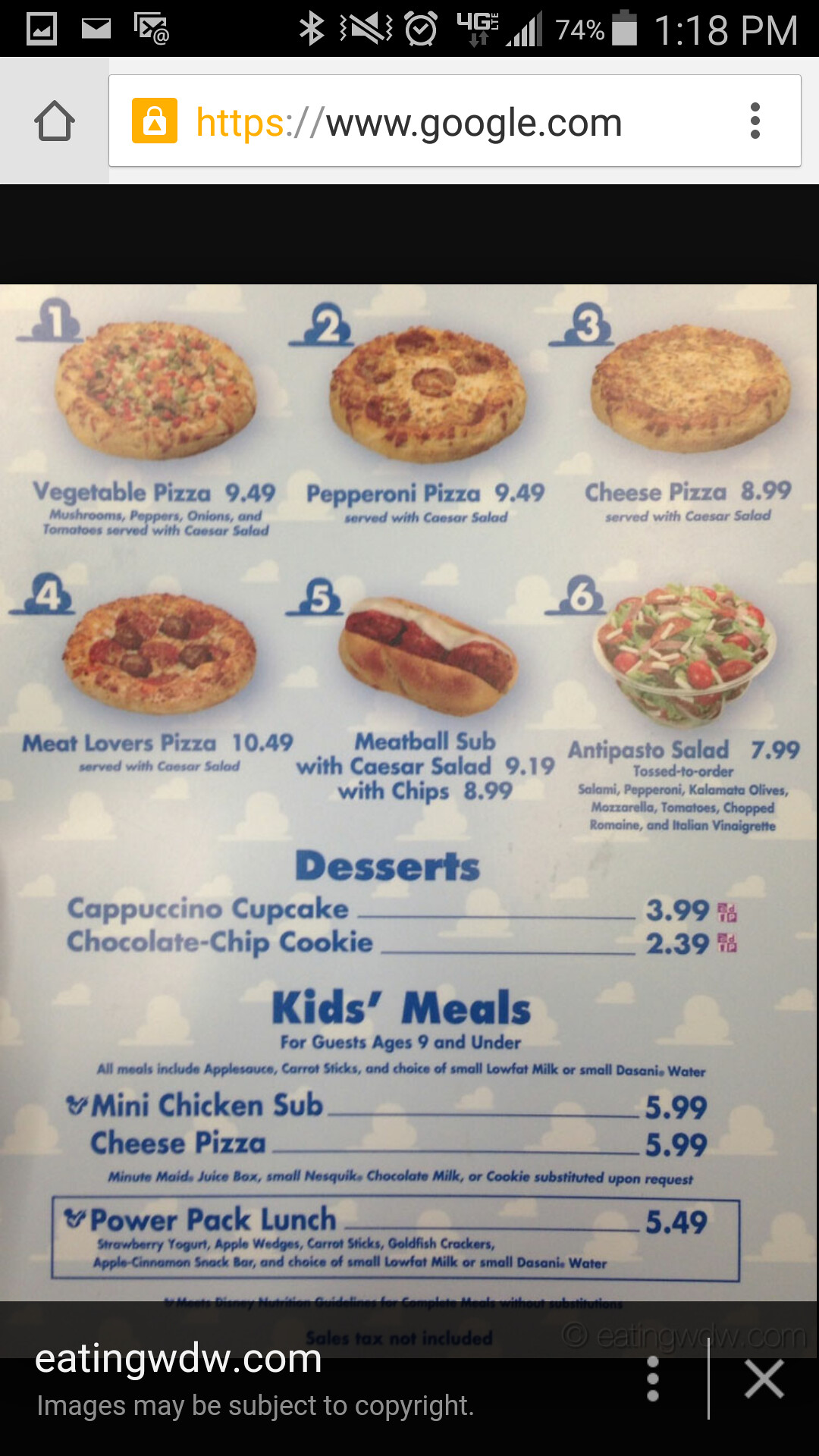In the image, you can see a meticulously arranged food menu featuring a variety of items, each accompanied by an image and a price. The top section of the menu showcases three pizzas: 

1. **Vegetable Pizza** priced at $9.49.
2. **Pepperoni Pizza** priced at $9.49.
3. **Cheese Pizza** priced at $8.99, which is served with a cheddar salad.

Below these, the numbered items continue from 4 to 6:

4. **Meat Lovers Pizza** priced at $10.49.
5. **Meatball Sub** served with a caesar salad and chips, listed at two prices: $9.19 and $8.99.
6. **Antipasto Salad** priced at $7.99, which includes detailed ingredients like pepperoni and tomatoes.

Further down the menu, there's a section dedicated to desserts, featuring:

- **Cappuccino Cupcake** for $3.99.
- **Chocolate Chip Cookie** for $2.39.

The kids' menu includes:

- **Mini Chicken Sub** for $5.99.
- **Cheese Pizza** for $5.99.
- **Power Pack Lunch** for $5.49.

All these items are set against a whimsical background featuring cartoon-like clouds, adding a playful touch to the menu display.